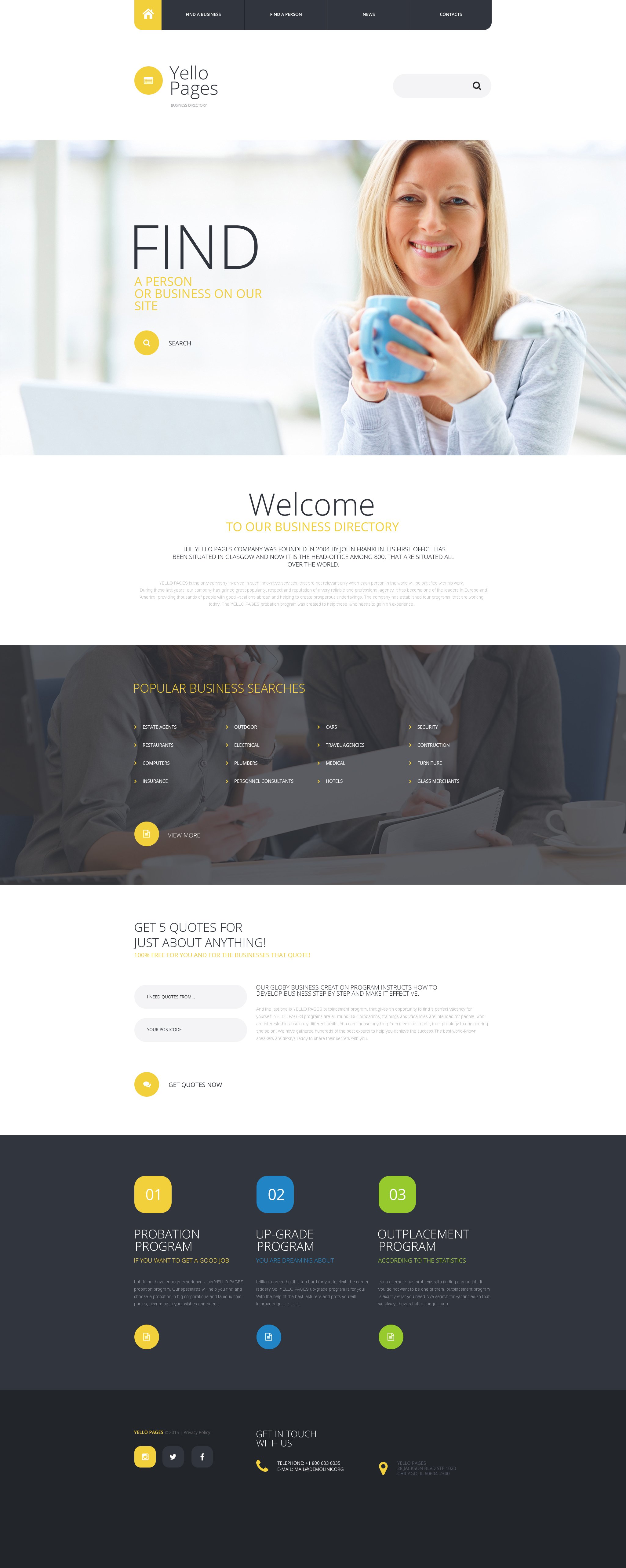The image displays the Yellow Pages website. In the upper left-hand corner, the Yellow Pages logo is prominently featured, with "Yellow" spelled out as "Y-E-L-L-O" in black font, and "Pages" situated directly underneath. Adjacent to the text is a yellow circle emblem. To the right of the logo, almost centrally aligned, is a search bar. Directly beneath this is a wide image that spans from left to right, depicting a cheerful woman with blonde hair seated at a desk. She is holding a blue coffee cup with both hands and smiling. In the lower right-hand corner of the image, the edge of a lamp is visible. To the left of the woman, there is text in black that reads "Find a person or business," followed by the words "on your site" in yellow. Beneath this image, there is a welcome section that reads, "Welcome to our business directory." Below this is a section labeled "Popular Business Searches."